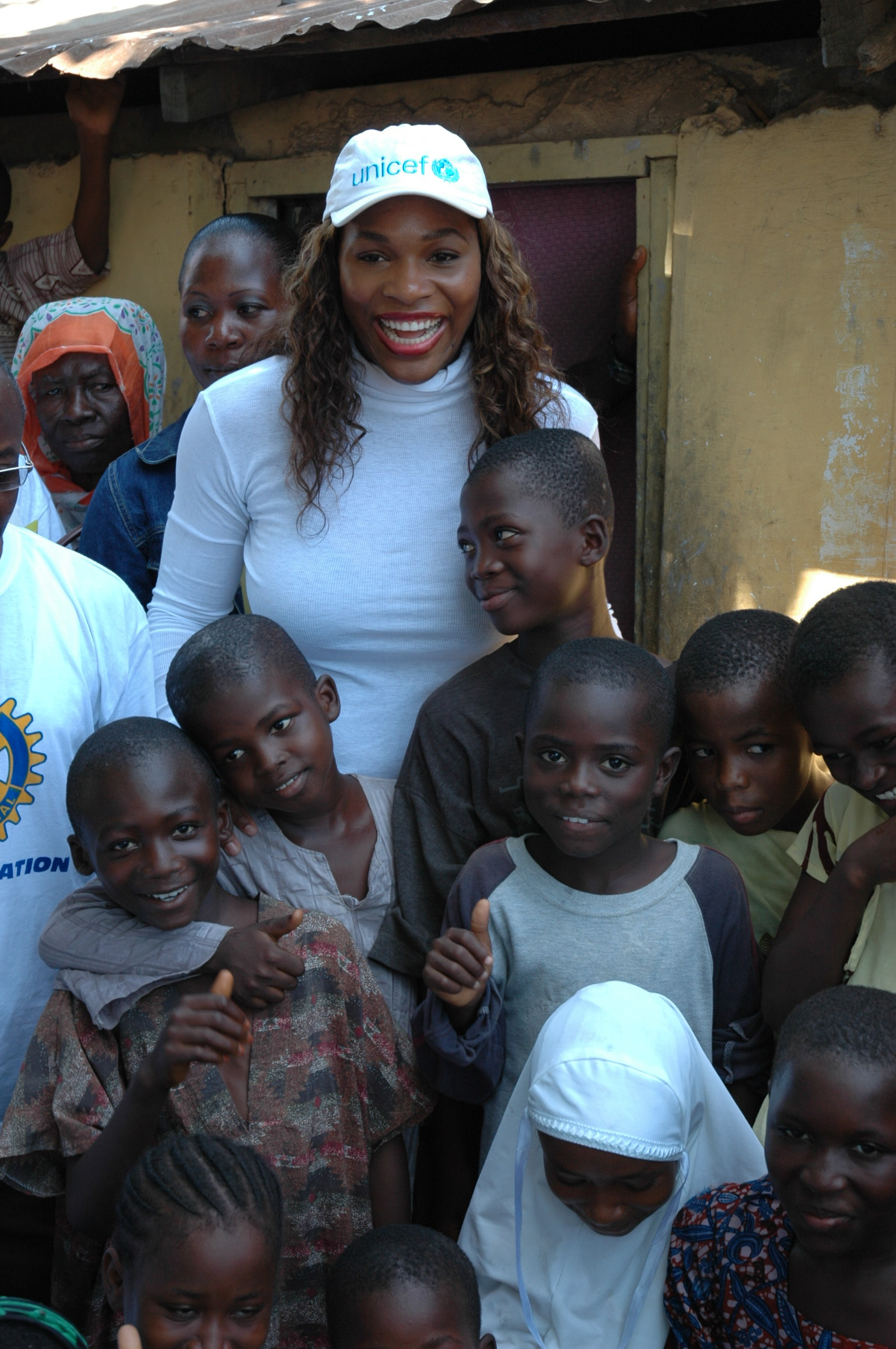The image captures a lively and heartwarming scene set in an African village. At the center, a smiling woman with a radiant grin, wearing red lipstick and a white turtleneck, stands out. Her curly, wavy hair cascades down to her chest. She appears to share a joyous moment with a group of people around her. The rustic backdrop features a rundown shack-like building with a corrugated tin roof, hinting at the simplicity of the setting.

Surrounding the central figure are various individuals, each adding to the vibrant tapestry of the scene. To her left, an older gentleman in a white T-shirt sports a symbol reminiscent of the rotary logo with blue and yellow spokes. Nearby, women wear distinctive head coverings adorned with floral patterns and solid orange designs. Another woman's hair is neatly pulled back into a bun, wrapped in what seems to be a blue jean jacket material.

In front of this diverse group stand several smiling children. Some boys are seen hugging each other, while others look in different directions, adding to the candid nature of the photograph. Among them, a little girl in a flowery shirt and a boy peeking from the side contribute to the overall sense of community and warmth. The bright, sunny day further illuminates the joyous atmosphere of this culturally rich and engaging scene.